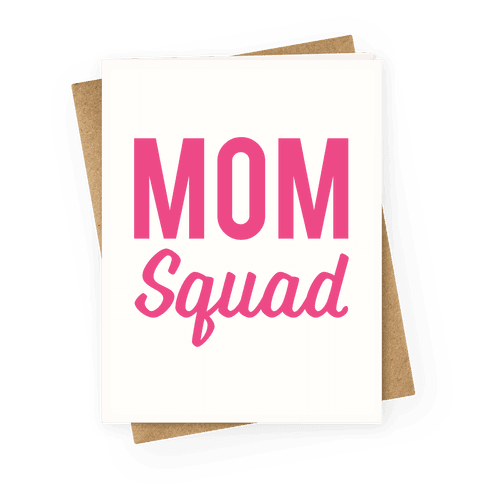This image features a design with a solid white background. Central to the composition is a white rectangular card tilted slightly to the left, resting at a modest angle. The card showcases bold, hot pink text. The top half of the card reads “MOM” in large, all-caps, thick font, occupying about 20% of the card's area centrally. Below, in a smaller, more delicate cursive font, the word “Squad” is displayed, with a capitalized 'S' and the remaining letters in lowercase. Both words are centered, offering a balanced appearance with equal white space above and below the text. Beneath this white card is a light brown rectangular piece, possibly cardboard or an envelope, positioned at a slight angle, exposing its corners and adding a layered dimension to the visual. The entire arrangement rests neatly on the pristine white background, creating a clean and organized look.